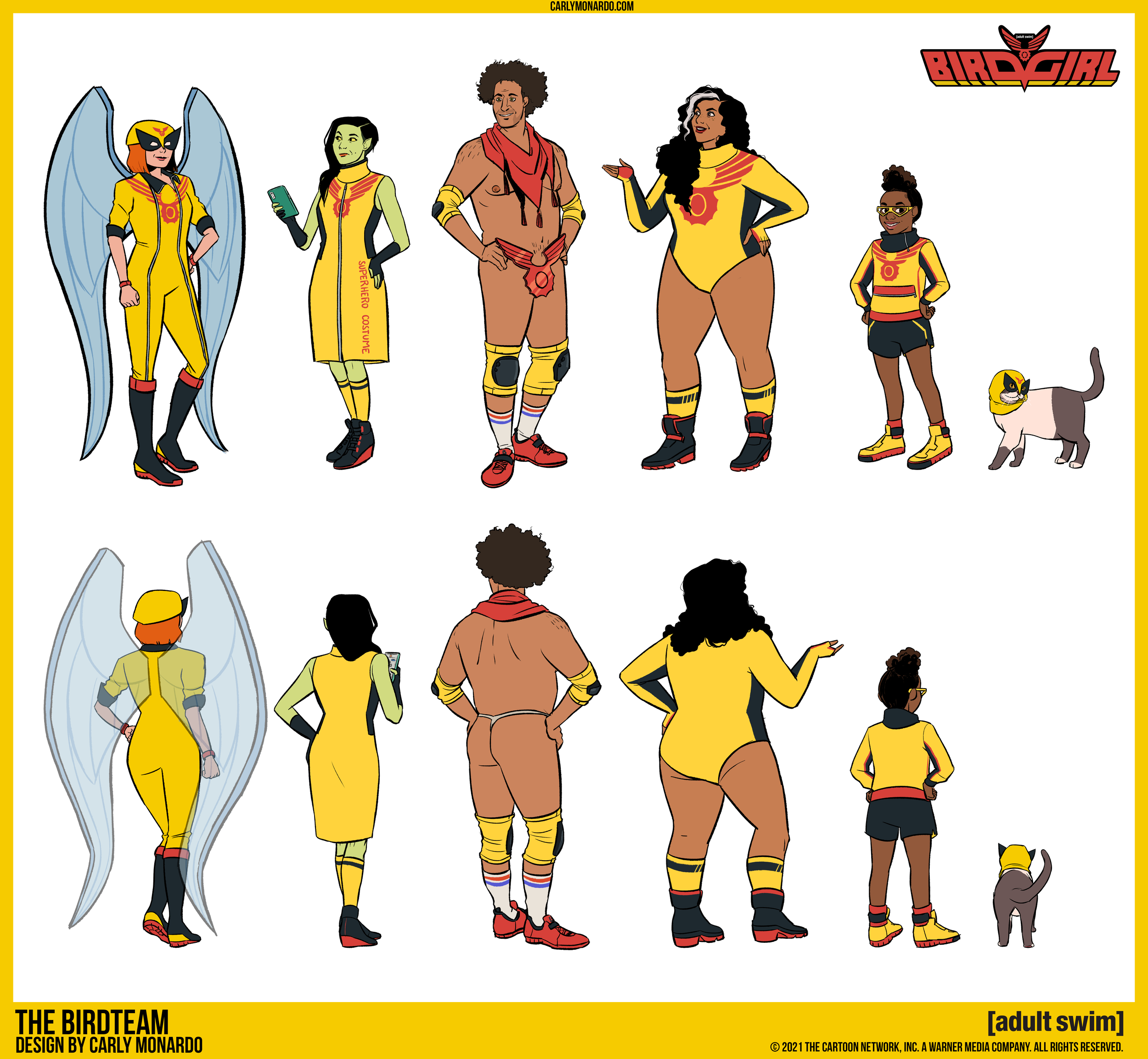The image is a promotional picture for the show "Bird Girl," showcasing a team of superheroes called "The Bird Team," designed by Carly Monardo. The picture is divided into two rows: the top row features six characters facing the viewer, while the bottom row shows these same characters facing away.

On the far left of the top row is a female superhero dressed in a yellow jumpsuit and mask, with large grayish-blue wings extending from her back. Beside her stands another female character in an orange dress, black gloves, and holding a cell phone, distinguished by her black hair. Next to her is a green-skinned woman with long black hair, also wearing a yellow outfit. Following her is a muscular male hero with a red bandana, brown skin, minimal clothing, and red metallic symbol over his lower region along with yellow knee and elbow pads. To his right is a bulky female character in a yellow suit, followed by a smaller African American child wearing a yellow shirt and black shorts or pants. The row ends with a distinctive white-and-gray cat donning a yellow cap, notable for its brown body and white stripes with a golden mane resembling a lion's.

In the bottom right corner of the image, the Adult Swim logo is prominently displayed, indicating the network associated with the show. The title "Bird Girl" appears in red lettering in the top right corner, accompanied by a symbolic emblem.